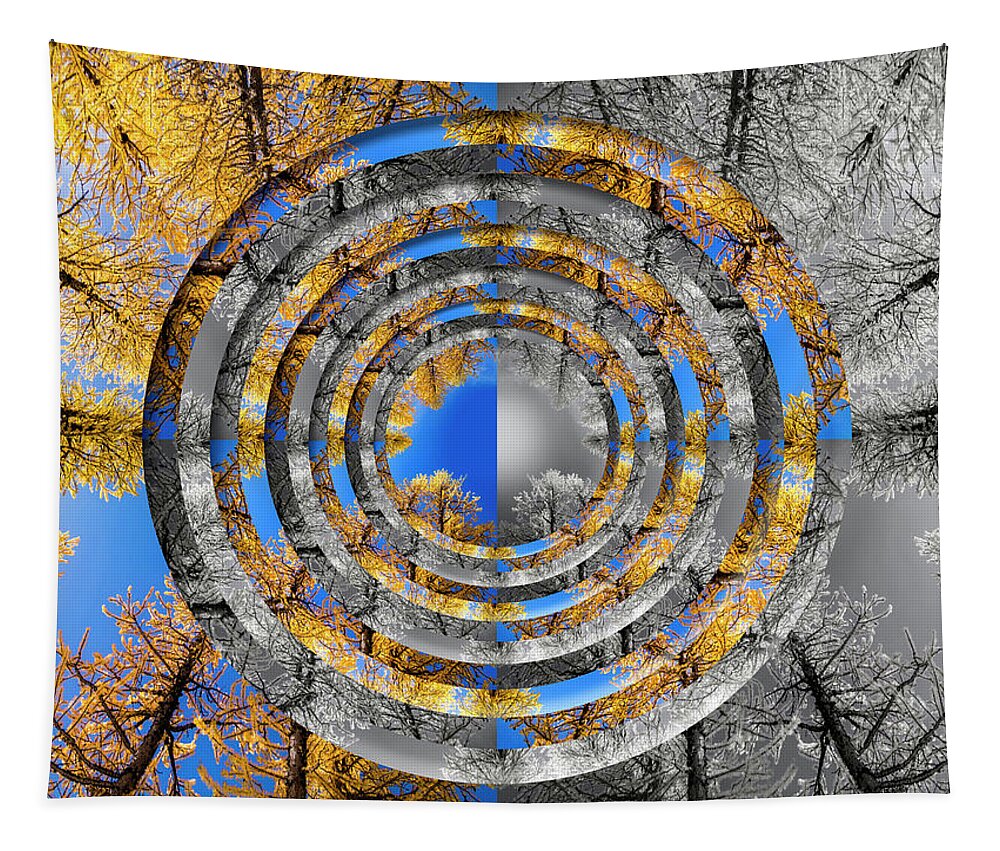The image showcases a rectangular printed blanket pinned at the top two corners to a white background, causing a slight curve from its weight. The central focus of the image is the blanket, featuring an intricately designed print that merges a half-colored and half black-and-white photograph of trees taken from a ground-up perspective. The color section on the left side of the blanket reveals a vivid blue sky and yellow leaves, while the right side displays a grayscale version of the same scene. A distinctive circular pattern spirals out from the center, alternating between the black-and-white and colored sections, creating an interlocking, trippy visual effect that blurs the boundaries between the two halves.